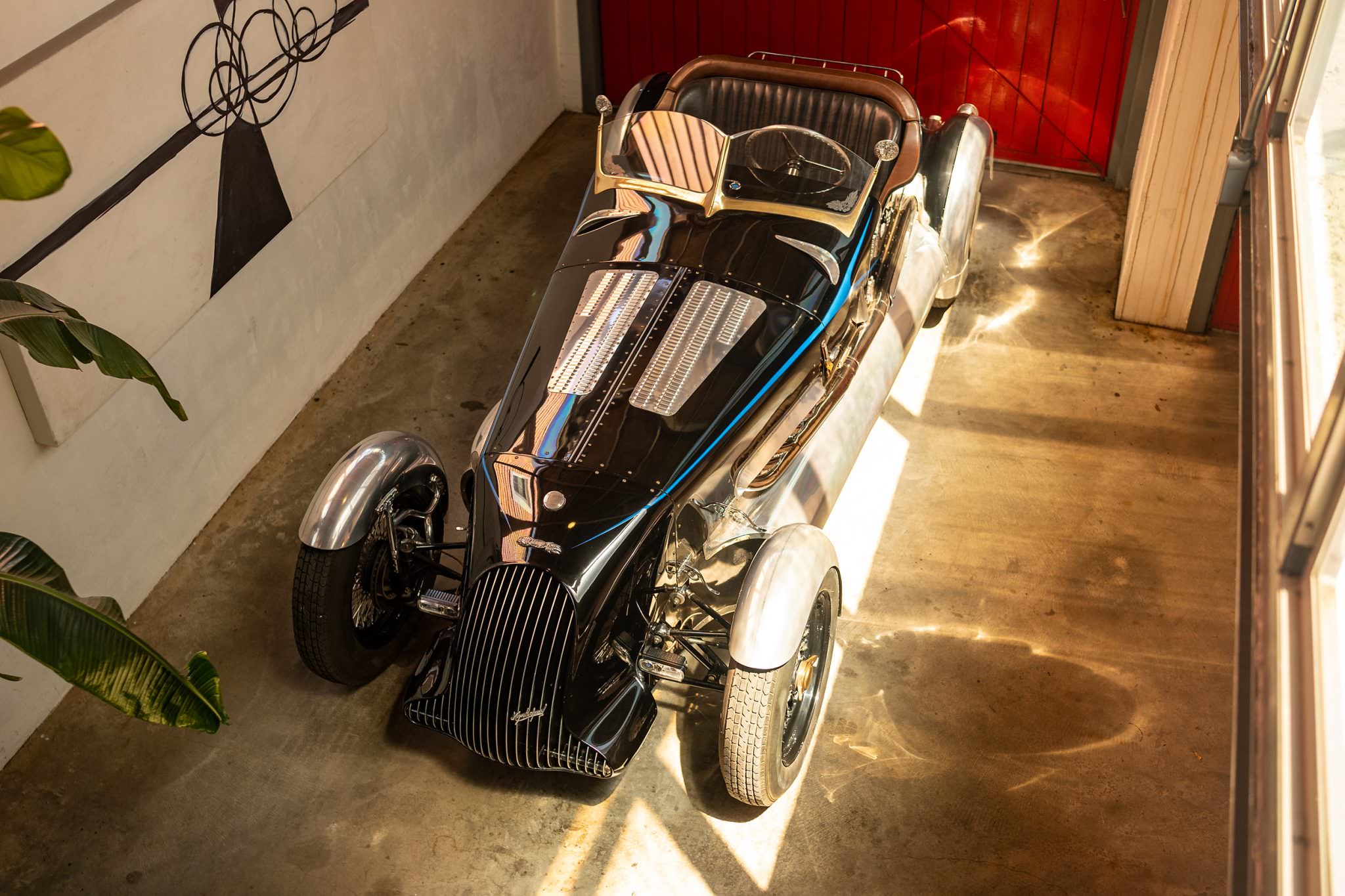This color photograph features a classic, yet contemporarily styled, soapbox derby car reminiscent of those raced by children with their fathers from the 1930s to the 1950s. The sleek, old-fashioned race car is a two-seater without a roof, primarily ivory-colored on the sides with a strikingly shiny black top that reflects a hint of blue. It has a distinctive contemporary grille with stylish gold lines and smaller headlights, while the tires evoke the 1940s era. The car is positioned diagonally in a small garage-like space, parked on a concrete floor stamped to resemble wood. The background features a red shiplap wall, an ivory white wall, and large windows on one side, allowing sunlight to stream in and illuminate the car. The decor includes a potted plant, contemporary black-and-white artwork, and an abstract painting, adding a touch of modernity to the otherwise vintage scene.